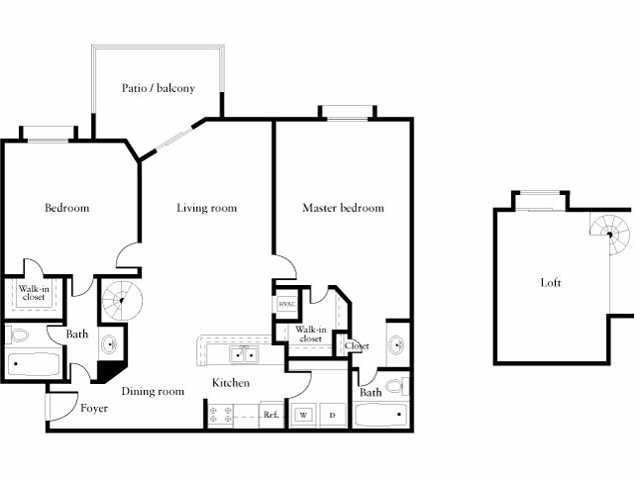This architectural design of a house features a comprehensive layout divided into distinct sections. The main structure, a large square, is delineated with various labeled areas, each serving a specific purpose. 

At the top of the design, a spacious patio/balcony is designated, offering an outdoor area for relaxation. On the left-hand side of the plan, there is a bedroom. The center of the design houses the living room, which serves as the heart of the home. To the right of the living room, a master bedroom is marked, providing a larger private space.

The bottom portion of the layout includes the dining room and foyer, indicating the entrance and main eating area of the home. Adjacent to these spaces is the kitchen, complete with detailed notations showing the locations of major fixtures such as the bathtub, toilet, and other amenities.

In the far left corner, there is a small square labeled "Bath," and nearby, additional squares mark a walk-in closet and another bath area, emphasizing the ample storage and convenience facilities.

Off to the left side of the main structure, a small isolated square is labeled "Loft" (L-O-F-T). Although detached from the main square, it includes its own design details, featuring a pinwheel symbol within the square, possibly indicating a decorative or functional element. 

Overall, this detailed architectural design thoughtfully maps out the various living spaces, providing a clear understanding of the house's layout and functionality.